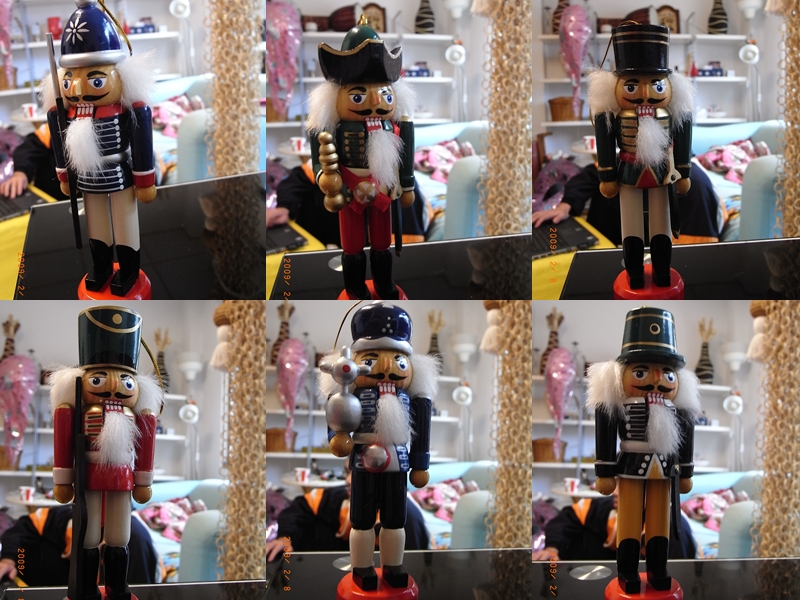This is a vibrant and detailed collage comprising six color photographs of wooden holiday nutcrackers. The nutcrackers are arranged in two rows of three, each facing the camera, allowing for a clear view of their intricately decorated fronts. Each nutcracker sports a light blue military uniform with subtle variations in their decorations, including differing hat styles such as a floral-patterned helmet, a naval officer's hat, a tall top hat, a gold-decorated hat, an oval-shaped blue and silver hat, and a bucket-shaped hat with gold embellishments. Their faces are uniformly adorned with painted eyes, mustaches, white hair, and white goatees.

The background of each photograph depicts a cozy bedroom setting with white shelving and various pink and blue objects, providing a glimpse into a lived-in space. A white chain-like column is visible along the right side of each photo, adding a unique structural element to the background. The images are slightly backlit, casting a shadow over the front of the nutcrackers and creating a subtle contrast that highlights their detailed features. The overall collage presents a charming and festive visual narrative without any accompanying text or printing, emphasizing the artistry and variety of the nutcracker figures against the consistent backdrop.